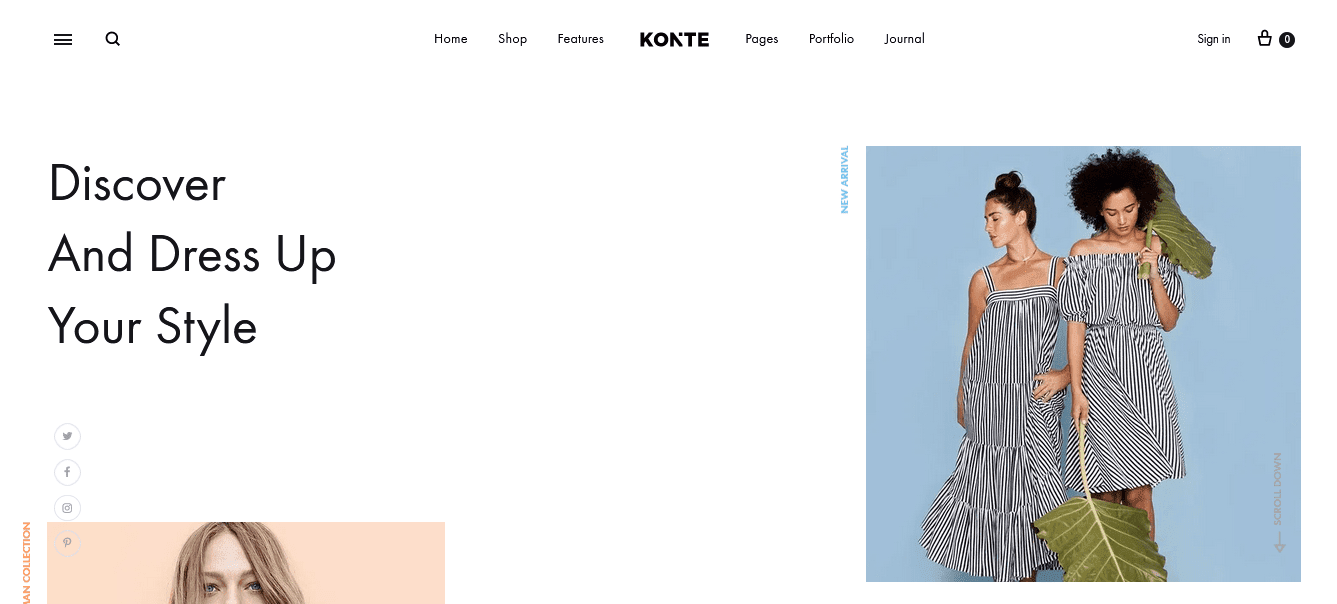The image displays a web page with a navigation bar at the top. The bar features three horizontal lines on the left, followed by a magnifying glass icon. Next to these icons are lightly outlined ovals with menu items labeled "Home," "Shop," an unclear word, "K-O-K-T-E" brand name (correctly "K-O-N-T-E"), another unreadable word, "Portfolio," and "Journal." On the far right of the bar are a "Sign In" option, a lock icon, and a round black dot with white details.

Below the navigation bar, in larger print, the text reads "Discover" on the first line, "Dress Up" on the second line, and "Your Style" on the third line, all in black font. 

Next, there is the top portion of a rectangle with a pink background displaying an image of a lady, only visible down to her nose. To the left, icons for social media platforms like Twitter and Facebook are visible. On the right side of the page, there is a blue square featuring a photograph of two women wearing black and white striped dresses, one of whom is holding very large green palm leaves.